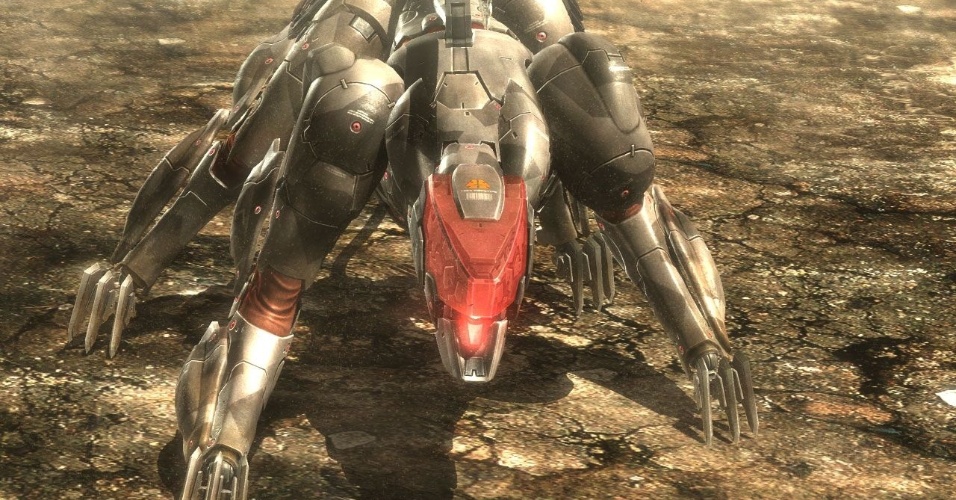The image is a screenshot from a video game, showcasing a mechanical, four-legged creature with a menacing stance. The creature, resembling a robotic dog, has a silver metallic body and is positioned in an aggressive, bent-over attack posture. Each of its four legs ends in sharp metallic claws, suggestive of its readiness to strike. Its head features a prominent red face shield, substituting for a traditional face, and a possible dark orange symbol can be observed on its forehead, adding to its ominous appearance. The background sets the scene on a dark, rocky surface, resembling volcanic rock, although the graphics give an illusion of texture despite being flat. The overall ambiance of the image is dark and gritty, emphasizing the creature's mechanical and hostile nature.